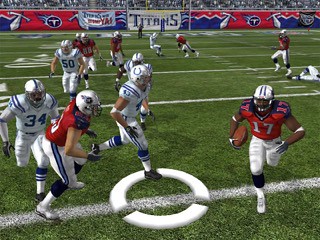A high-resolution screenshot from an NFL video game, possibly from the 2K series, depicts an intense moment on the football field. The setting is a sprawling stadium filled with spectators, their excitement palpable. Prominently visible in the upper section of the image is a wall adorned with various graphics, including a white sign that reads "Titans" in bold letters. The meticulously detailed football field below is a rich green, marked with crisp white yard lines that add to the realistic feel of the game. Scattered across the field are virtual football players, predominantly dressed in sharp white uniforms, but a few are donned in vivid red. Notably, in the lower right corner of the screenshot, an African American player in a dynamic red uniform can be seen sprinting, capturing the essence of the action-packed gameplay.